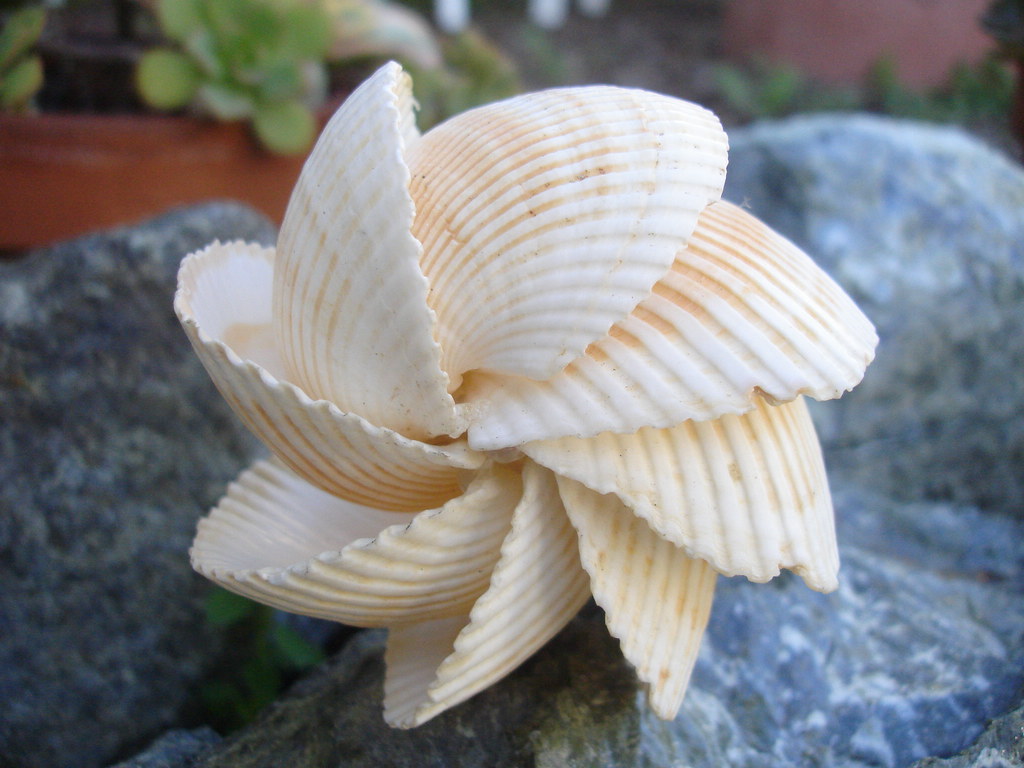This photograph captures a meticulously arranged group of eight similarly sized, cream-colored seashells, each accented with orange-tinted lines. The seashells, all of the same species, are placed in a spiral pattern reminiscent of a pinwheel or circular flower, with their bases converging at the center and creating a flowing, overlapping sequence. The intricate shell formation rests on three large, rough-hewn stones in shades of black, gray, and white, which provide a contrasting backdrop to the delicate arrangement. In the blurred background, a medium-brown wooden table is adorned with two potted plants featuring green leaves, and in the upper right corner, additional greenery and part of a red structure are partially visible. The shells and stones occupy the central focus of the image, effectively highlighting the intricate artistry and natural textures present.